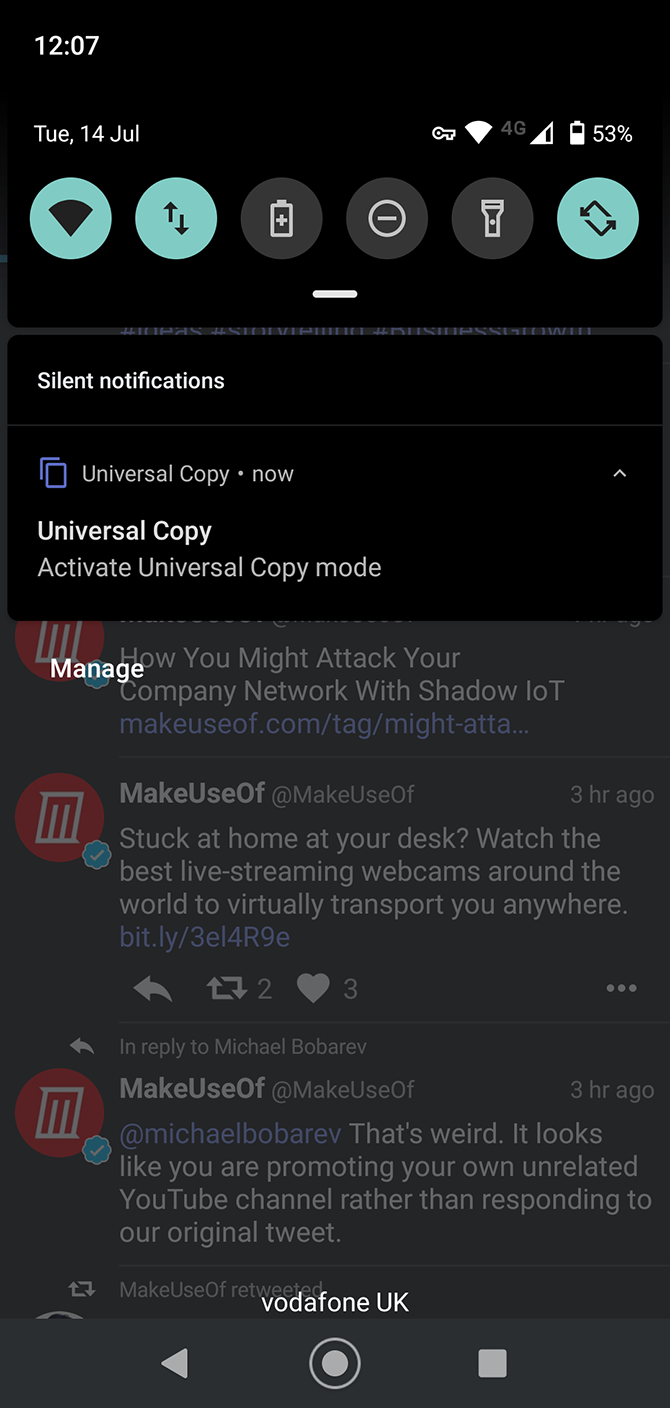The image captures a detailed view of an Android phone with its notification area pulled down, revealing both notifications and quick settings. One prominent notification is from an app called "Universal Copy," suggesting the activation of a mode to copy any text on the screen. The quick settings show several toggles: Wi-Fi is active, there is an icon with up and down arrows likely indicating data usage, a battery saver mode, Do Not Disturb mode, auto-rotate feature, and a flashlight. In the background of the phone screen, the user is browsing Twitter, specifically viewing the "MakeUseOf" Twitter account, which is known for tech-related content. One visible tweet from the account reads, "That's weird, it looks like you are promoting your own unrelated YouTube channel."